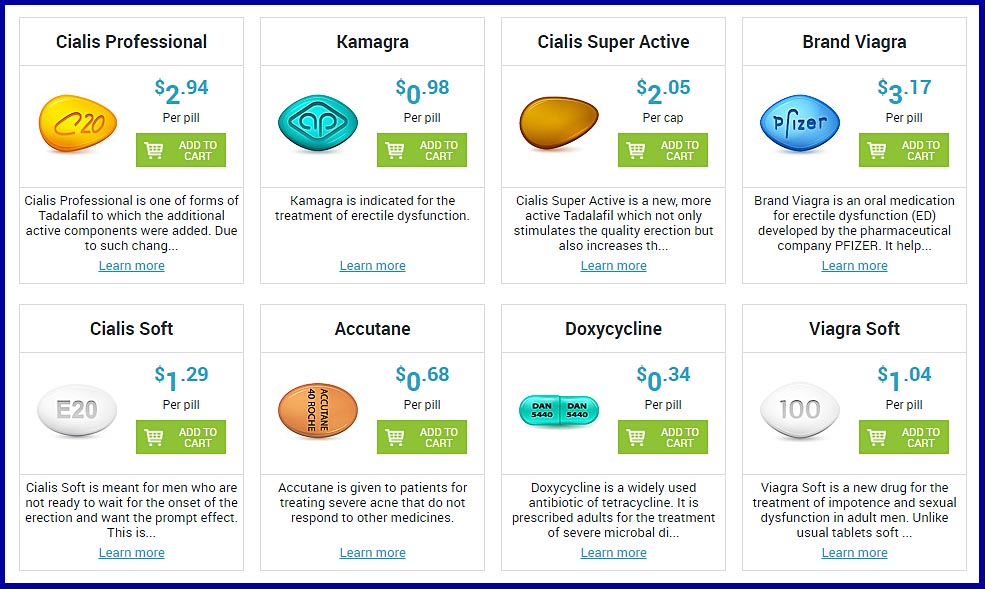Here is a detailed and cleaned-up caption for the described image:

---

The screenshot is rectangular with a blue border and predominantly features a white background, containing eight distinct columns of information. 

1. **Cialis Professional:** 
   - **Image:** Depicts a yellow tablet with the imprint "C20."
   - **Price:** $2.94 per pill.
   - **Add to Cart:** Features a green rectangular button labeled "Add to Cart."
   - **Description:** "Cialis Professional is a form of Tadalafil enhanced with additional active components, aimed at improving efficacy." Below the description, a "Learn More" hyperlink provides further details.

2. **Camagra:**
   - **Image:** Shows a bluish-green tablet with the letters "AP" imprinted on it.
   - **Price:** $0.98 per pill.
   - **Add to Cart:** Displays a green rectangular "Add to Cart" button.
   - **Description:** "Camagra is indicated for the treatment of erectile dysfunction." A "Learn More" hyperlink is available beneath the description.

3. **Cialis Superactive:**
   - Description and details aligned similarly to the previous listings with essential info like price, and an "Add to Cart" button.

4. **Brand Viagra:**
   - Description and details continue consistent layout with the essential pricing and purchase options as mentioned above.

In the second row:

5. **Cialis Soft:**
   - Continues with a similar structure of image, price, and "Add to Cart" button alongside the product description.

6. **Accutane:**
   - Maintains the same format with its relevant details displayed similarly.

7. **Doxycycline:**
   - Follows the established pattern of image, pricing, and description with purchase options.

8. **Viagra Soft:**
   - Displays consistent design elements and information as noted in the other columns.

---

Each column's layout includes the product name, an image of the pill/tablet, the price per pill, an "Add to Cart" button, and a brief description with a "Learn More" link for additional information.